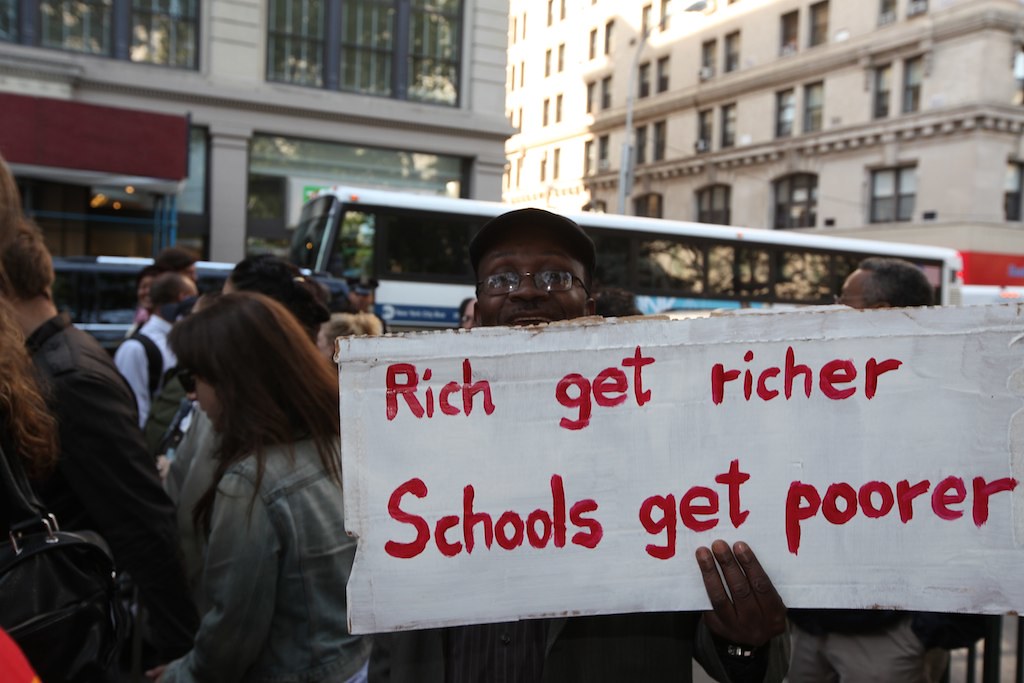A black man wearing a baseball hat and glasses stands prominently in the foreground, holding up a white cardboard sign painted in red with the message "Rich Get Richer, Schools Get Poorer." He holds the sign firmly in his left hand, with three fingers on top and his thumb and pinky behind it; a watch is also visible on his wrist. The man appears to have a slight smile but is focused on conveying his message about the education system. 

Behind him, there are several other people walking by, seemingly going about their day without joining the protest. A large transit bus with a white top and numerous windows can be seen in the background. The setting is a bustling city street, framed by tall buildings with many windows on one side and smaller shops on the other. The sun shines on one of the buildings, highlighting the urban environment of the scene.